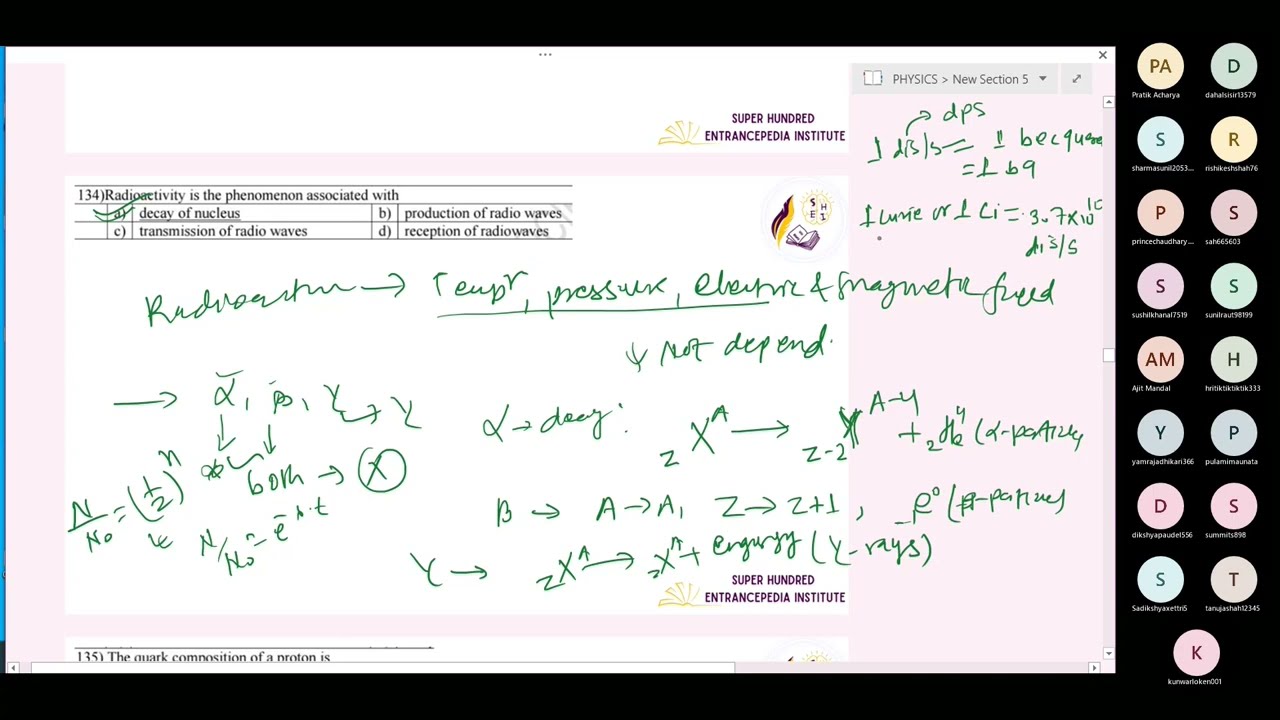This detailed image captures a digital screen in the middle of a live streaming session, resembling a shared screen often seen in educational reviews or Zoom sessions. The central focus is a multiple-choice physics question projected in handwritten and typed text, set against varied backgrounds of white and pink. The header reads "Super 100 Intraspedia Institute," with a mention of "Physics, New Section 5" in the top right. The question posed is, "Radioactivity is the phenomenon associated with," followed by four options: A) decay of nucleus, B) production of radio waves, C) transmission of radio waves, and D) reception of radio waves. A pen marking highlights option A, indicating it as the correct answer. Below the question, handwritten notes and equations in green pen further explain the topic.

The right-hand column of the screen serves as a roster of attendees, featuring tiny circles filled with initials like 'PA' and 'D,' symbolizing the active participants in the session. These circles are color-coded in light hues such as greens, yellows, pinks, and blues. Despite their abundance, the names small and difficult to decipher. The entire screen is encased within a dual-layered border—black on the outer layer and pink on the inner—with portions of text and snippets of written explanations peppered across the display, some in purple with accompanying yellow emblems. All around, the screen presents a densely packed and colorful tableau of collaborative learning, focused squarely on dissecting and understanding the physics question on radioactivity.